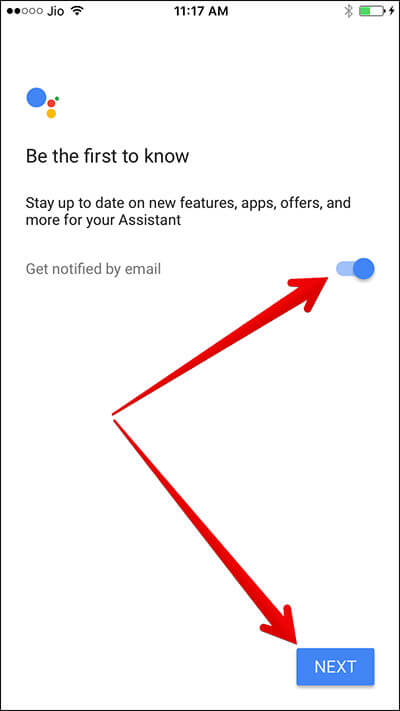The screenshot depicts a section of a JIO web page, captured on a smartphone. In the top-left corner of the screen, there are five circular icons, with the left two highlighted. Next to these icons, "JIO, JIO" is displayed, followed by a strong Wi-Fi signal icon. Centrally positioned is a timestamp reading "11:17 AM." To its right, there are icons for Bluetooth and battery, with the battery indicator showing approximately half charge. Below these, there appears a sequence of dots: a large blue dot, a small green dot, a red dot slightly larger than the green, and an orange dot of similar size to the red dot.

Underneath these elements, black text reads: "Be the first to know. Stay up to date on new features, apps, offers, and more for your assistant." Below this text, there is an option labeled "Get notified by email." Two arrows are present—a diagonal upward arrow starting about a quarter from the left of the page pointing to a toggle button, which is switched on, and a downward diagonal arrow pointing to a "Next" button, indicating where users can proceed. The webpage is identified as part of the JIO platform.